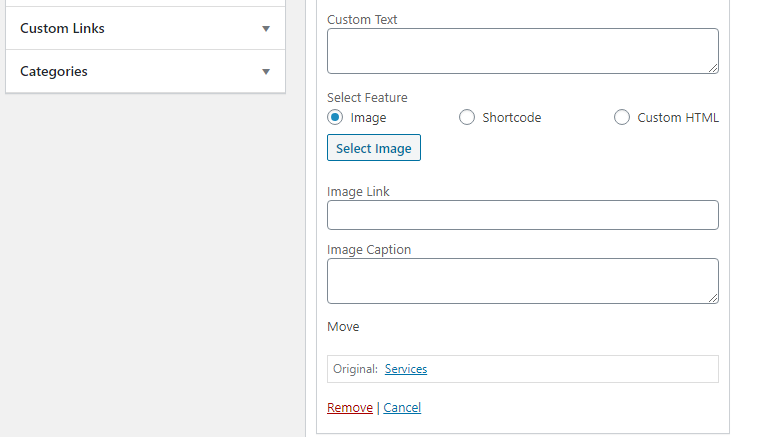This image is a screenshot of an unidentified web interface. The image is horizontally oriented, being wider than it is tall, and primarily text-based without any photographic elements or depictions of people, animals, plants, or vehicles.

On the left side of the screenshot, there is a light gray area featuring two drop-down menus at the top, set against a white background. These menus are labeled "Custom Links" and "Categories."

The right side of the image has a white background and includes multiple textual elements:
- The heading "Custom Text" followed by an empty input field for user input.
- A selectable radio button labeled "Select Feature Image."
- Options for "Shortcode" and "Custom HTML."
- Additional text links: "Select Image," "Image Link," "Image Caption."
- Functional options such as "Move," "Original Services" (highlighted in some manner), "Remove" (displayed in red text), and "Cancel" (highlighted in blue text).

There are no graphical or visual elements beyond text and user interface components present within the screenshot.